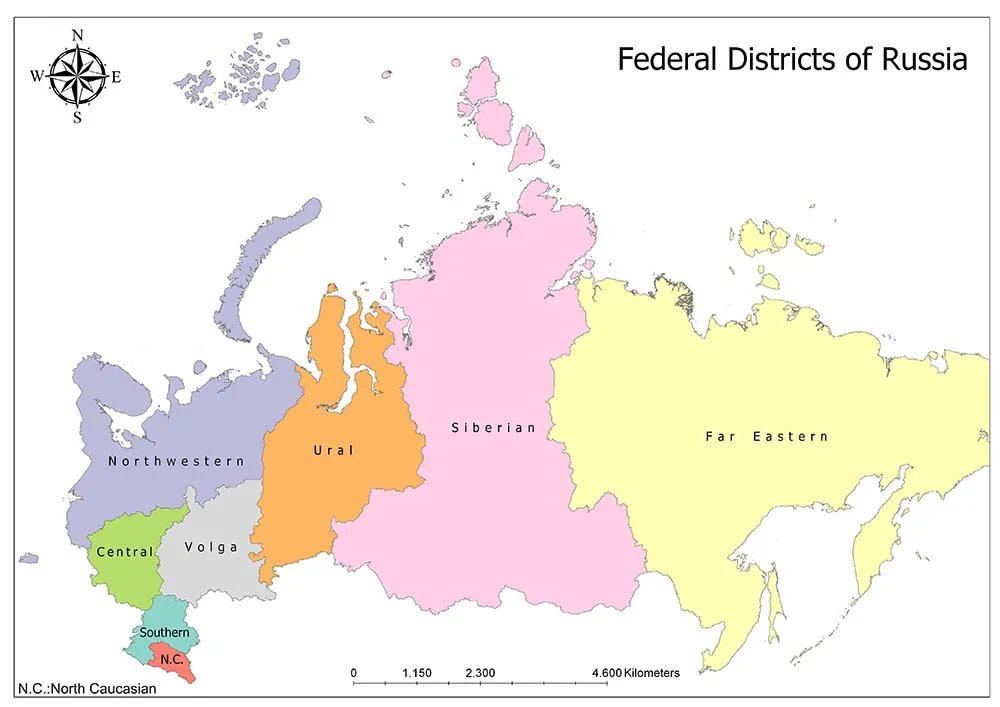This horizontal map titled "Federal Districts of Russia" features a star-shaped compass in the top left corner, indicating North, East, South, and West. On the right side, each federal district is color-coded against a simple, detail-free background. The largest district on the far right is the yellow-marked Far Eastern. Moving leftward, the pink district labeled Siberian follows, which is narrower in the middle and expands towards the edges. Adjacent and further left, the orange-colored Ural district is about half the size of the Siberian district. To the west of Ural lies a blue district labeled Northwestern, which includes a larger landmass and several smaller islands. Directly below Northwestern, lies a small green district called Central, and to its right is the gray-colored Volga district. Below these, two diminutive districts are positioned side-by-side; the teal-colored Southern district is situated above the coral-colored NC (North Caucasian) district, which is the smallest in size.